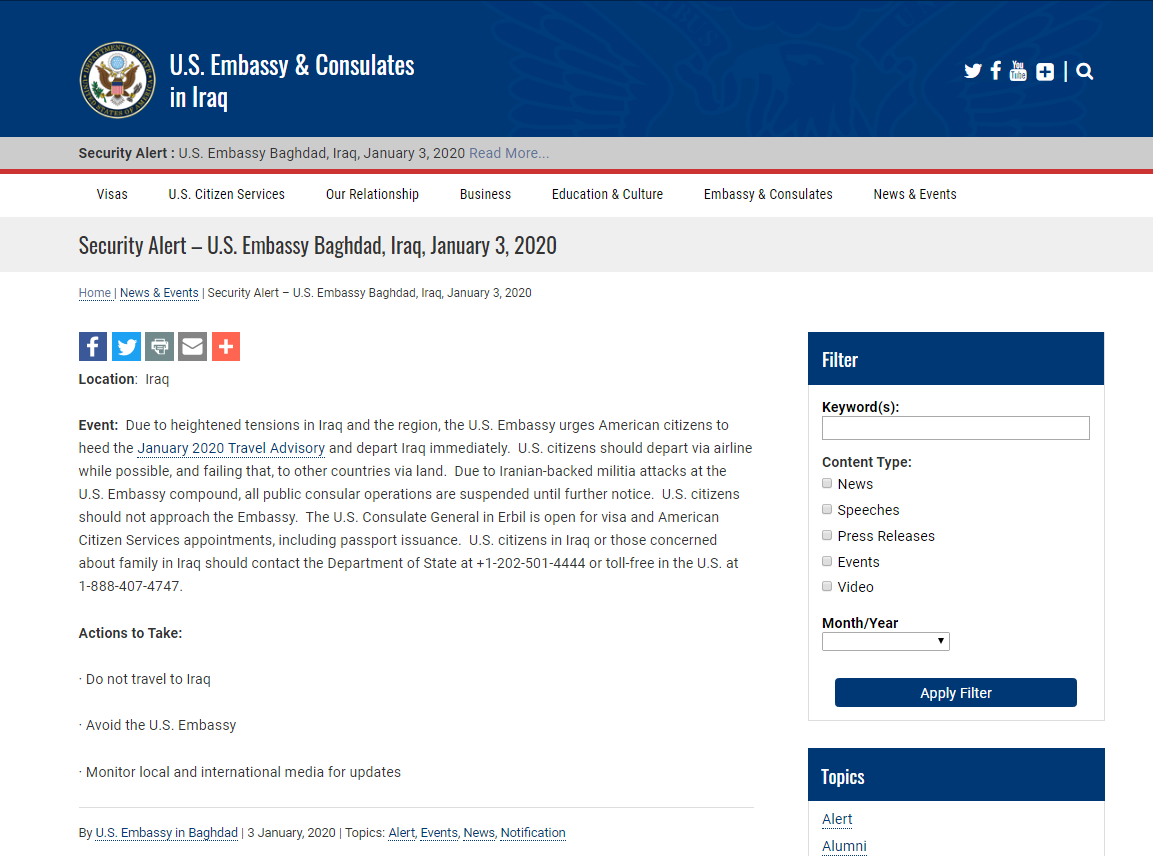A comprehensive screenshot of the U.S. Embassy and Consulates in Iraq website, prominently featuring a blue header bar at the top. On the left side of the header is the official United States government seal, followed by the text "U.S. Embassy and Consulates in Iraq." To the right, social media icons for Twitter, Facebook, YouTube, alongside a plus sign and a magnifying glass symbolizing additional options and search functionality. Below the header, a grey notification bar announces a "Security Alert, U.S. Embassy Baghdad, Iraq, January 3rd, 2020," with a prompt to read more.

The main navigation menu follows, with categories including Visas, U.S. Citizen Services, Our Relationship, Business, Education and Culture, Embassy and Consulates, and News and Events. A secondary notification bar reiterates the security alert. The detailed content section beneath shows a path breadcrumb reading Home > News and Events > Security Alert > U.S. Embassy Baghdad, Iraq, January 3rd, 2020 > Location: Iraq. A paragraph elaborates on the alert, stating that due to increased tensions in Iraq and surrounding regions, the U.S. Embassy advises American citizens to follow the January 2020 Travel Advisory and leave Iraq immediately. Additional advisory texts include actions to take such as avoiding travel to Iraq, steering clear of the U.S. Embassy, and monitoring local and international media for updates.

On the right side of the page, a sidebar widget allows visitors to filter content by keyword, content type (news, speeches, press releases, events, video), and time frame (month and year).